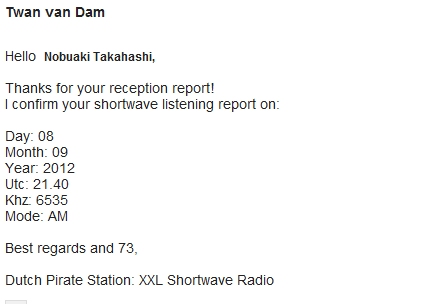The image depicts a small text document resembling an email or a short message, prominently featuring a white background with black text. At the top, the name "Tuan Van Dam" is printed in bold black text, followed by the greeting "Hello Nobuaki Takahashi" with the recipient's name also in bold. The body of the text reads: "Thank you for your reception report! I confirm your shortwave listening report on: day 08, month 09, year 2012, UTC 21:40, kHz 6535, mode AM. Best regards and 73, Dutch Pirate Station XXL shortwave radio." This document serves as a confirmation letter from Dutch Pirate Station XXL, verifying the receipt of a shortwave listening report from Nobuaki Takahashi.